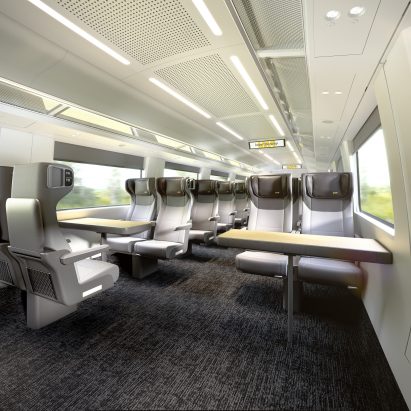This image captures the sleek, modern interior of a high-tech train. The setting is predominantly black, white, and shades of gray, contributing to an elegant atmosphere. The walls and ceiling are pristine white, adorned with numerous small dots that resemble speakers and accompanied by ample overhead lighting. Arranged in rows, the seating consists of sophisticated white and gray seats with dark gray headrests. On the left side of the image, there are two seats facing each other with a table in between, while the right side showcases forward-facing seats with individual tables. The tables are a light wood color, contrasting subtly with the overall monochromatic theme. The floor is covered in a black and gray carpet, adding to the refined ambiance. Large windows run along the sides, topped with gray window coverings that are pulled up, revealing a view of passing trees and a serene light blue sky outside. The motion blur through the frosted windows suggests the train is moving, lending a dynamic quality to the photograph. Signs are visible on the ceiling, though their details are blurred and indistinct. Overall, the image encapsulates the minimalist, high-tech elegance of this upscale train interior.